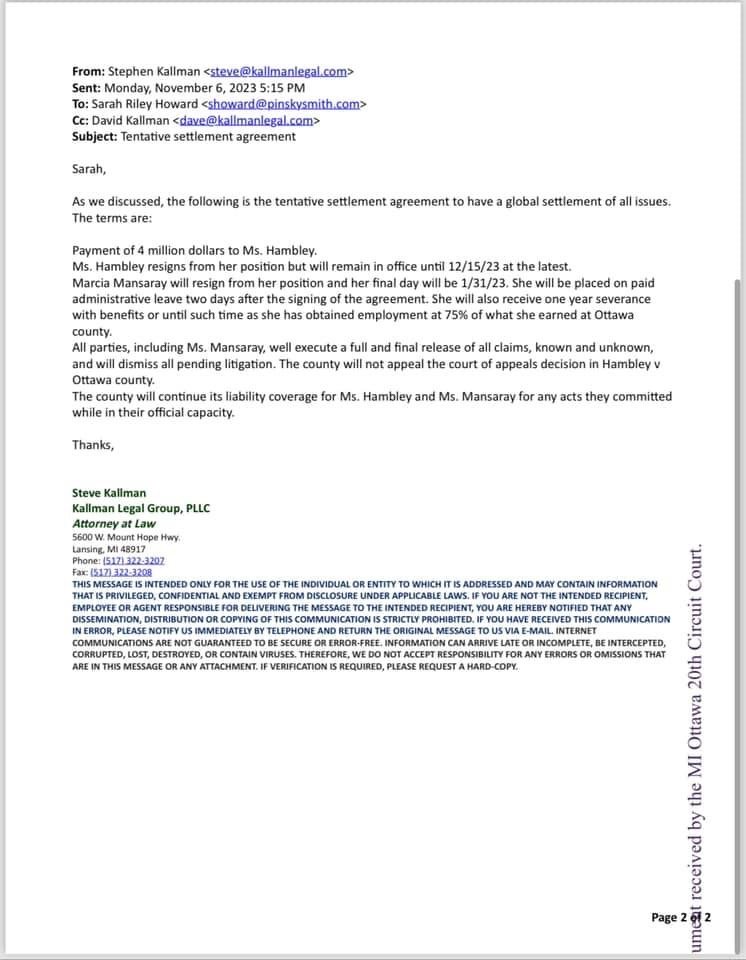Here is a cleaned-up and more detailed caption based on the provided text:

---

This detailed email, sent by Stephen Collman (steve@collmanlegal.com) on Monday, November 6, 2023, at 5:15 PM to Sarah Riley Howard (howard@picasvet.com) and C.C.'d to David Collman (dave@collmanlegal.com), outlines the terms of a tentative settlement agreement. The subject of the email pertains to a comprehensive global settlement involving all insurance terms.

The key points of the settlement include:

1. A payment of $4,000,000 to Ms. Hambly.
2. Ms. Hambly will resign from her position but will remain in office until December 15, 2023, at the latest.
3. Marsha Mansuray will resign from her position with a final date of January 31, 2023. She will be placed on paid administrative leave two days after the signing of the agreement. Additionally, she will receive a four-year severance of benefits or until she secures employment earning at least 75% of her Ottawa County salary.
4. All involved parties, including Ms. Mansuray, will sign a full and final release of all claims.
5. There will be a dismissal of all pending litigation by all parties.
6. The county will not appeal the Court of Appeals decision in the case of Ms. Hambly v. Ottawa County.
7. The county will continue to provide liability coverage for Ms. Hambly and Ms. Mansuray for any acts committed while they were in their official capacities.

The email concludes with a signature line that reads: "Thanks, Steve Collman, Legal Group, PLC, Attorney at Law."

---

This caption captures the essence and details of the described situation, providing clear information about the settlement terms and parties involved.